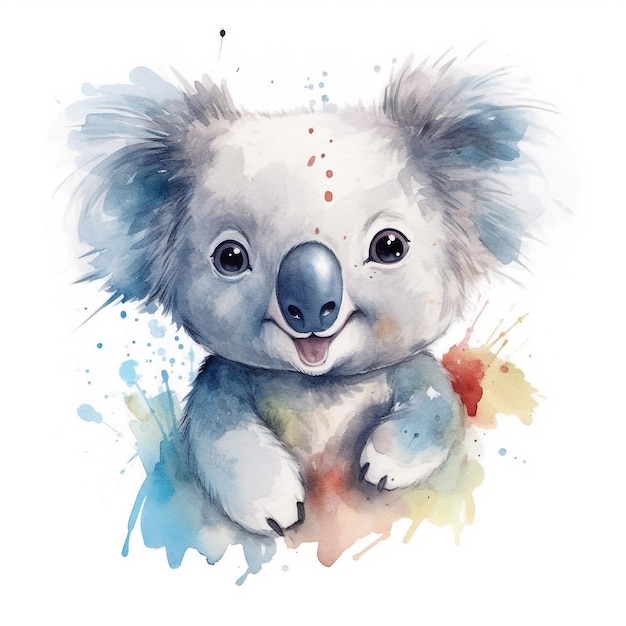The image is a square watercolor painting of a baby koala set against a white background. The koala is depicted from the chest up in a sitting posture, directly engaging viewers with wide, expressive eyes. Its striking features include a large blue nose, a happy smile with a hint of a pink tongue, and two black lines on each paw representing toenails. The koala's fur is illustrated in varying shades of white, gray, and blue, with the bluish tones more prominent on its ears and body. Notably, the eyes are encircled by different hues, with one eye having a blue ring and the other a gray ring, adding depth to its innocent gaze. The painting is accentuated by vibrant splatters of colors: blue and orange prominently marking the koala’s forehead, and larger splotches of red, yellow, and blue around and below its body, enhancing the whimsical and playful feel of the artwork.